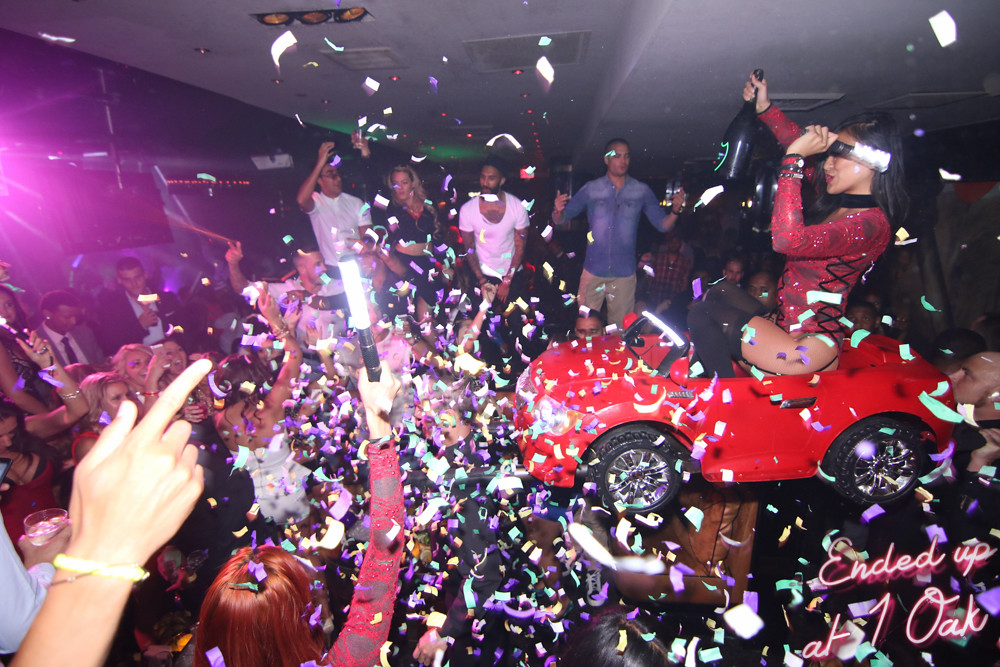The image captures an exuberant party scene inside what appears to be a nightclub, "One Oak," as indicated by pink neon-styled text in the bottom right corner. The atmosphere is filled with multicolored confetti—purple, white, and yellow—floating through the air, adding to the festive vibe. In the foreground on the right, a woman, dressed in a striking red long-sleeved leotard with black straps and thigh-high black boots, sits confidently in a red toy child’s car. She waves a light in one hand and holds a black bottle, possibly champagne, in the other. The image is alive with energy, as multiple people throughout the room face towards her, some with their hands raised, and many holding lights. The scene is set against a backdrop of a white ceiling and a black far wall, with purplish strobe lights creating an electric ambiance, possibly illuminating a dance floor to the left. The central group appears to be elevated on a platform, drawing attention as they revel in the confetti-filled celebration.